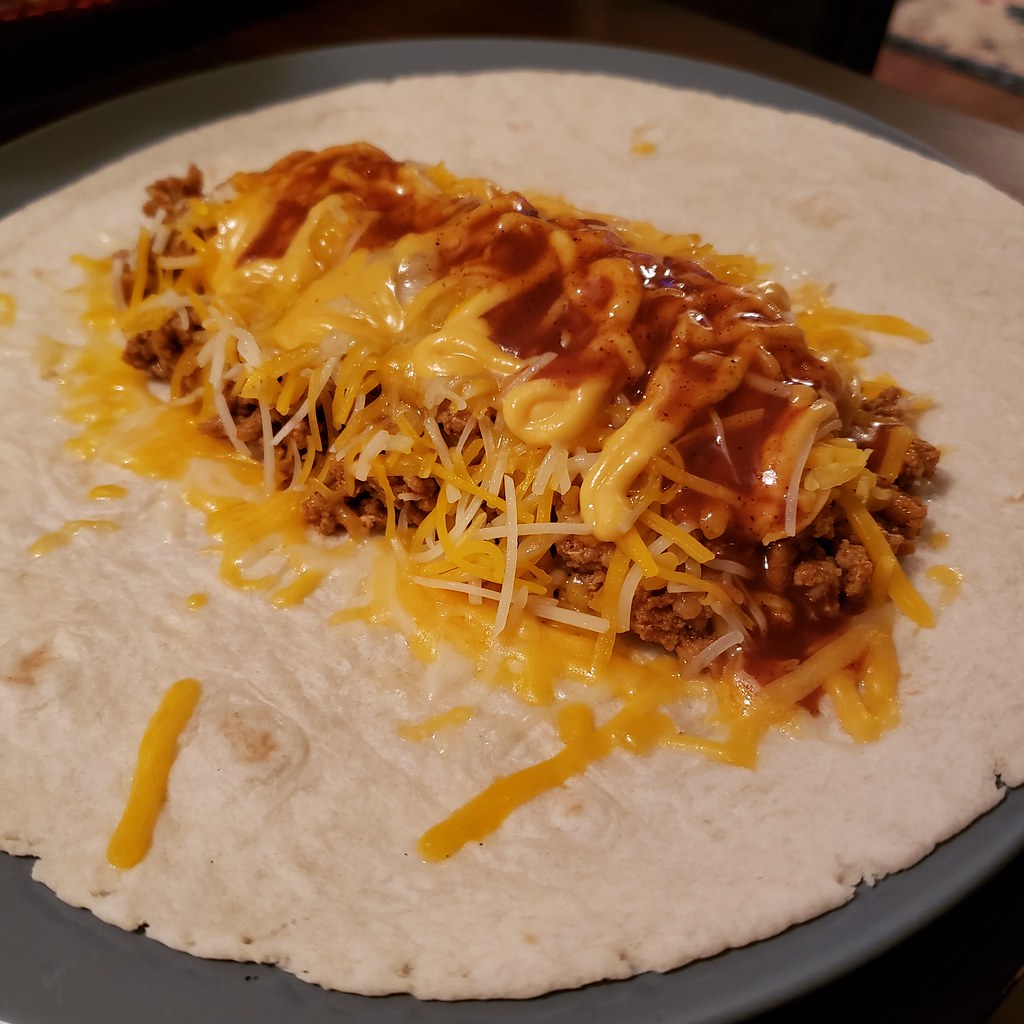This detailed close-up photograph captures an unrolled burrito laid flat on a gray matte plate, which rests on a brown wooden table with a glimpse of carpet in the background. The white flour tortilla serves as the base, and in the center, there is a linear arrangement of fillings. The bottom layer consists of ground meat, moist with its own juices, topped generously with shredded cheese. This is followed by a layer of nacho cheese sauce and a drizzling of hot red sauce. The scene suggests that the burrito is in the process of being folded, transforming from its open, flat state into a closed burrito ready to eat.